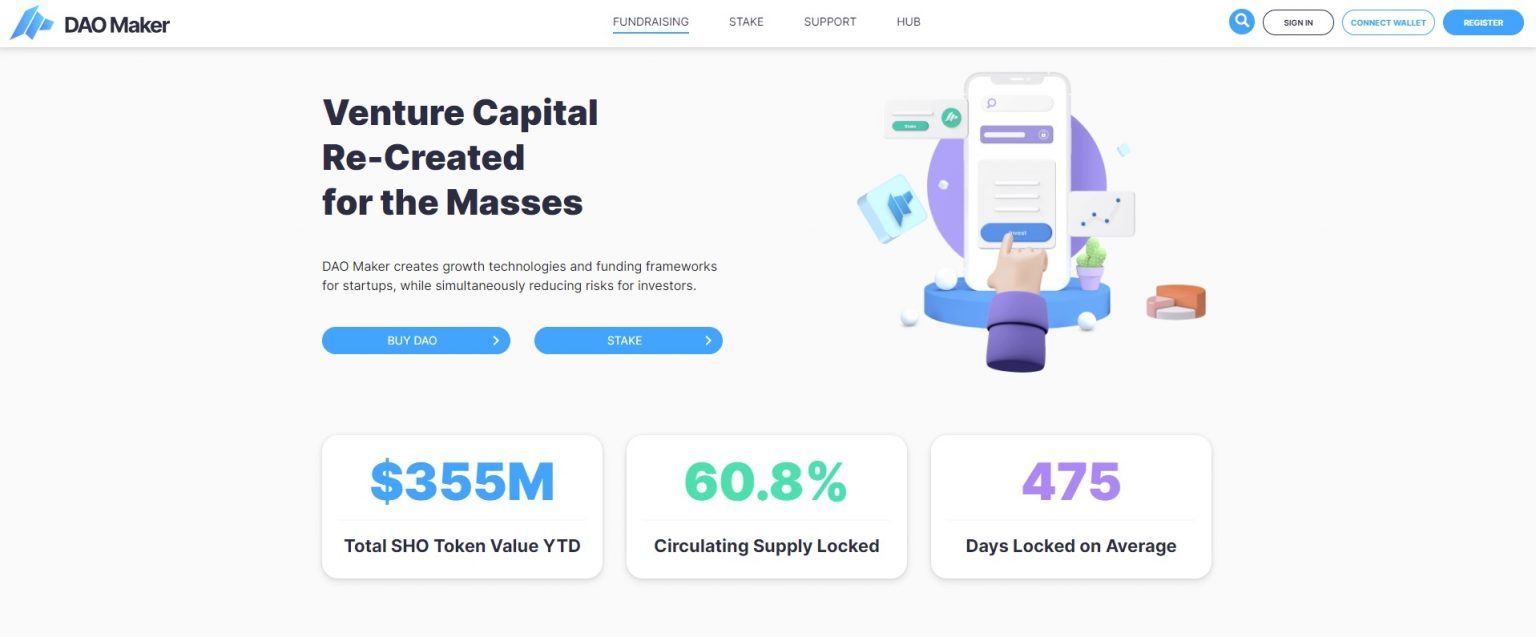**Website Caption for DAO Maker:**

The DAO Maker website features a sleek design with a very light grey background and prominent white navigation bar at the top. On the left side of this bar, the DAO Maker logo is displayed conspicuously, while the center houses four navigational menu options: Fundraising, Stake, Support, and Hub. Currently, the Fundraising page is active, indicated by a small blue line beneath it. On the right side of the navigation bar, there are icons for search, sign in, connect wallet, and register.

The main section of the page also maintains a light grey background. On the left, bold text announces "Venture Capital recreated for the masses." Below this, in a smaller font, it states "DAO Maker creates growth technologies and funding frameworks for startups while simultaneously reducing risks for investors." This is accompanied by two prominent blue buttons labeled "Buy DAO" and "Stake," followed by an animated icon of a hand pressing a phone button.

Beneath these elements are three adjacent white boxes that highlight key metrics. The first box displays "355 million total SHO token value year to date" with the figure "355 million" in blue. The second box states "60.8% circulating supply locked," and the third one shows "475 days locked on average."